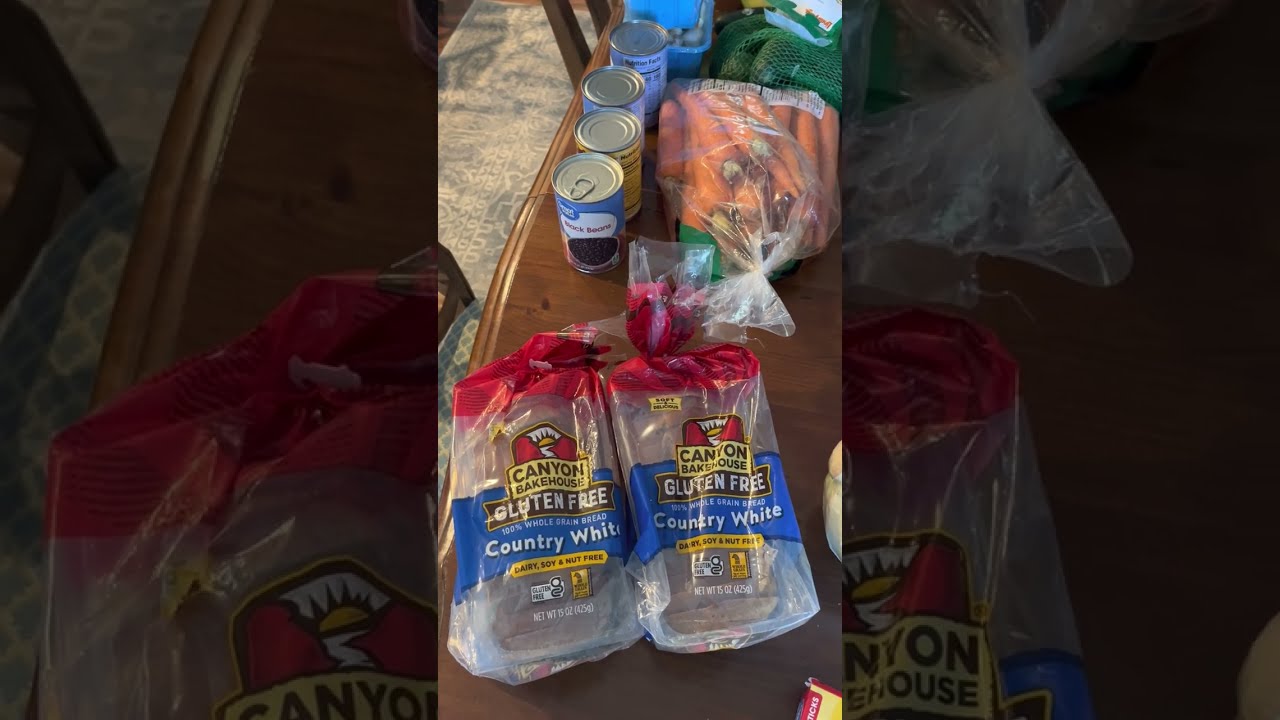The image captures an overhead view of a slightly curved, decorative wooden dining table, adorned with various grocery items. Dominating the foreground are two packages of Canyon Bakehouse gluten-free white bread, identifiable by their semi-transparent plastic packaging with a blue stripe. Behind the bread, four cans of food are arranged in a row, with the first can being a Great Value can of black beans clearly visible. To the right of the cans lies a transparent plastic bag filled with carrots, approximately a three-pound bag. Scattered further on the table are additional items, including bags possibly containing mushrooms and avocados, indicating a recent shopping trip, presumably from Walmart, given the presence of the store’s private labels on several items. The table is set against a zoomed-in, faded background image of the same scene, enhancing the central focus on the assortment of groceries arranged meticulously for an upcoming meal preparation.